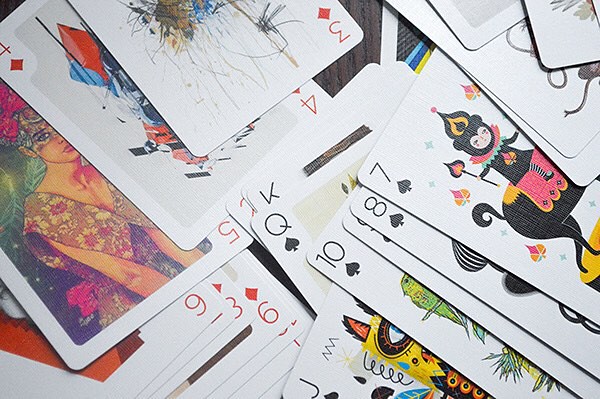This rectangular image features a spread of playing cards showcased with their numbers and suits facing upward. In the lower right corner, a row of cards is laid out, beginning with a Jack of Spades, which partially displays an image resembling a llama. Next is a 10 of Spades adorned with green birds. A mostly obscured card follows, likely another Spade. An 8 of Spades is visible with just some black lining peeking out, and a 7 of Spades captures attention with a peculiar illustration of a harlequin-like monkey figure riding a horse-like creature, wielding a scepter and donning a crown.

In the upper right-hand corner, there's a stack of playing cards, their faces concealed. Transitioning to the top and left corner, the 3 of Diamonds catches the eye with its intricate artistic design, followed by a 4 of Diamonds featuring a red, blue, and black motif. The 5 of Diamonds, in red, depicts a masked woman in an elaborate outfit. Beneath her, additional cards are stacked, but their numbers and images remain largely hidden.